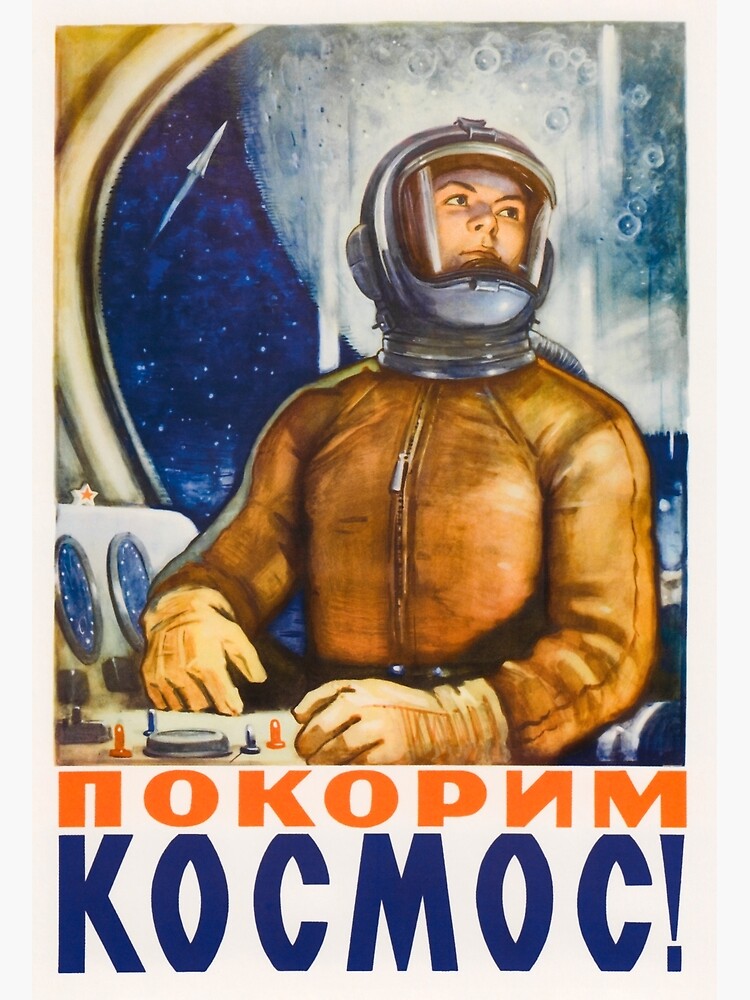This vintage-style movie poster features a male astronaut at the center, adorned in a rusty brown suit with tan gloves and a silver helmet with a viewfinder. He is positioned at a command console with his body facing forward, but his gaze is directed upwards to the right. The background showcases a large, prominent moon in the upper corner, along with a rocket shooting towards it against a dark blue, star-filled sky. Behind the astronaut, a window reveals this cosmic scene, enhancing the space setting. Sketchy art elements add a hand-drawn quality to the image. At the bottom of the poster, the Russian text "Н-О-К-О-Р-Н-М" in red and "К-О-С-М-О-С!" in blue emphasizes the movie’s theme. The entire poster is framed in white, contributing to its classic, retro aesthetic.